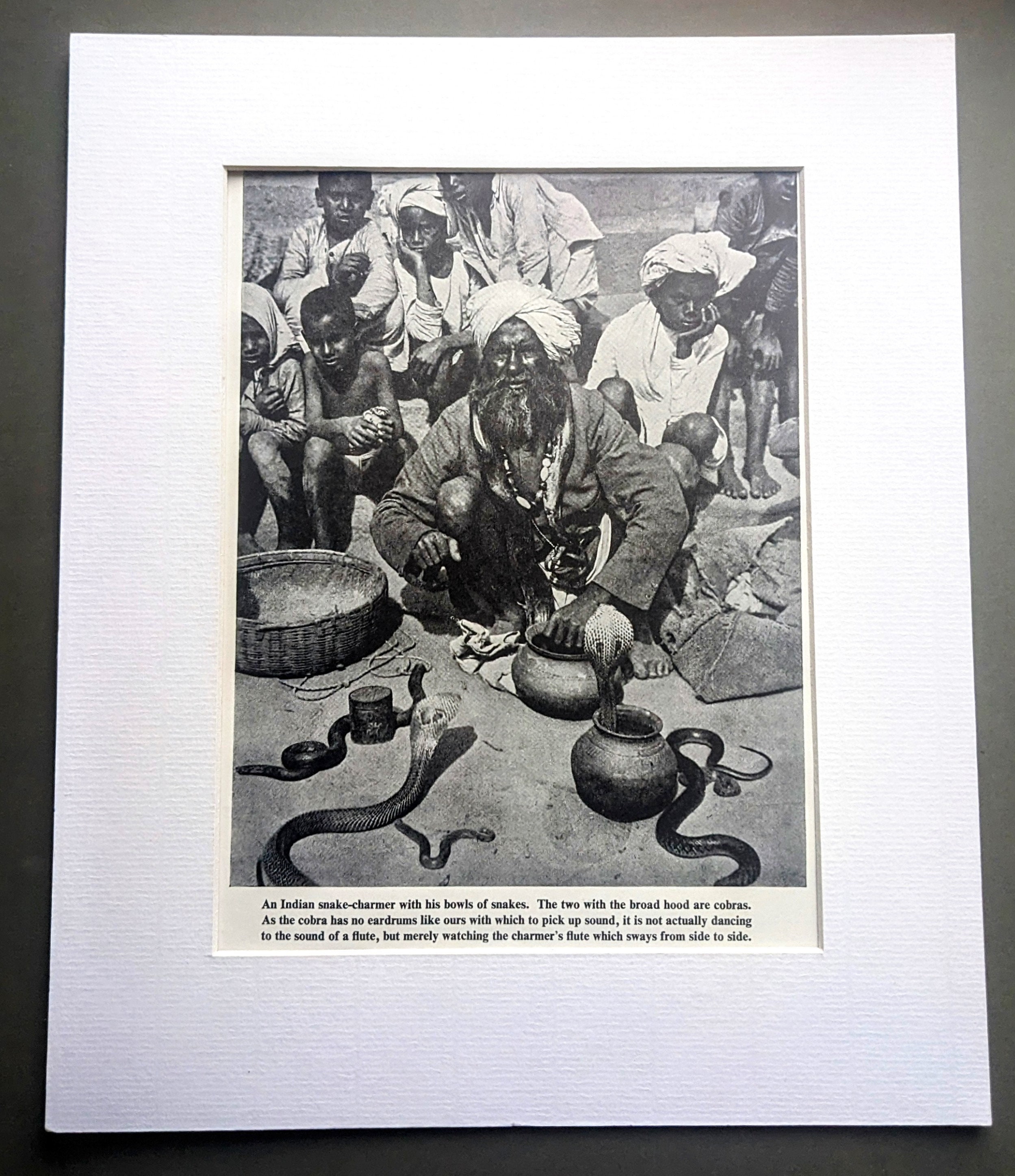This detailed description features a framed, black-and-white photograph in a white frame that rests against a dark gray surface. The photo, set elegantly within a black-bordered frame, showcases an elderly Indian man, identifiable by his turban and traditional attire, kneeling on the ground amidst an array of snakes. Several children, similarly attired, are seated behind him, attentively observing. The scene is enlivened by the presence of numerous snakes, including cobras with broad hoods emerging from pots in front of the man. Captivating the viewer, the text at the bottom of the photograph reads: "An Indian snake charmer with his bowls of snakes. The two with the broad hoods are cobras." Further text informs, "As the cobra has no eardrum like ours with which to pick up sound, it is not actually dancing to the sound of a flute, but merely watching the charmer's flute, which sways from side to side." Despite the frame's modest size, the rich details and traditional charm of the scene it encloses command significant attention.